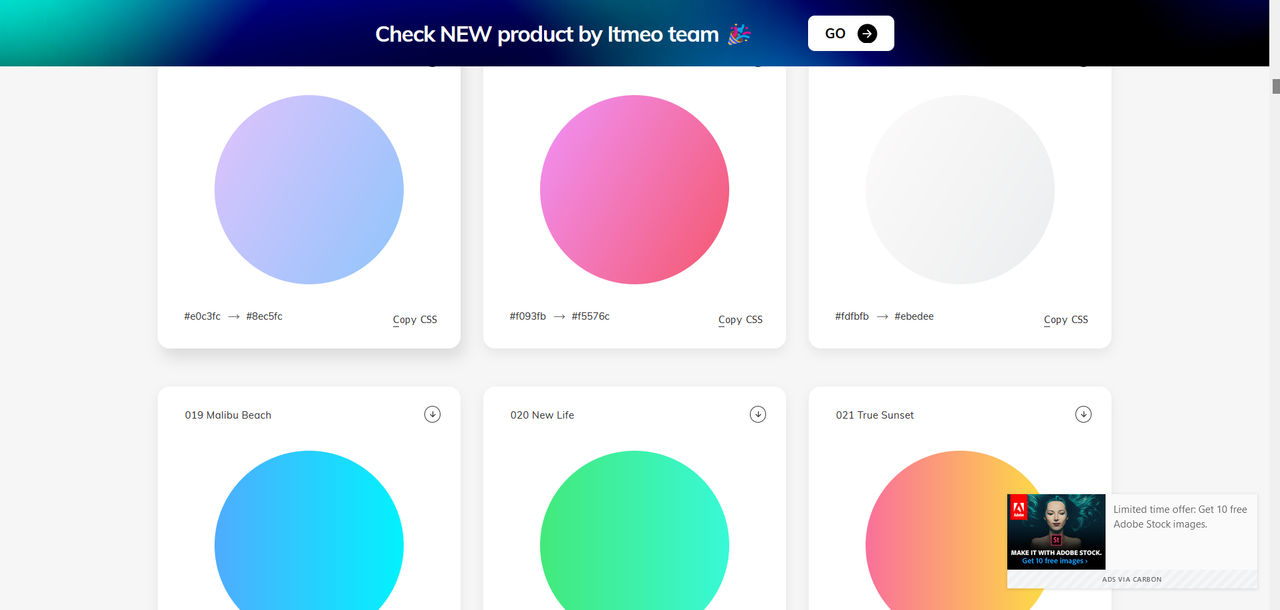The image showcases a vibrant and eye-catching display. At the top, there's a thick bar that transitions from aqua to blue and finally to black. Within this bar, the text reads "Check new product by ITMEO team," accompanied by an interactive "Go" button with an arrow.

Below this bar, there are nine squares arranged in a 3x3 grid. Each square contains a large circle, although the bottom three circles are partially clipped. The bottom row of squares includes a number ID and the text "Copy CSS," a feature also present in the top three squares.

In the upper left-hand corner of the middle row squares, the circles are labeled as "019 Malibu Beach," "020 New Life," and "021 True Sunset." The circles themselves display a range of colors: light blue, pink, and off-white, as well as gradients—blue to aqua, green lightening as it moves right, and pink transitioning to orange.

In the bottom right-hand corner of the image, there is an ad labeled "Ads via Carbon," which promotes a "Limited Time Offer" for 10 free Adobe Stock images, with accompanying text "Make it with Adobe Stock." It is unclear whether this ad is part of the main display or a separate, listed advertisement.